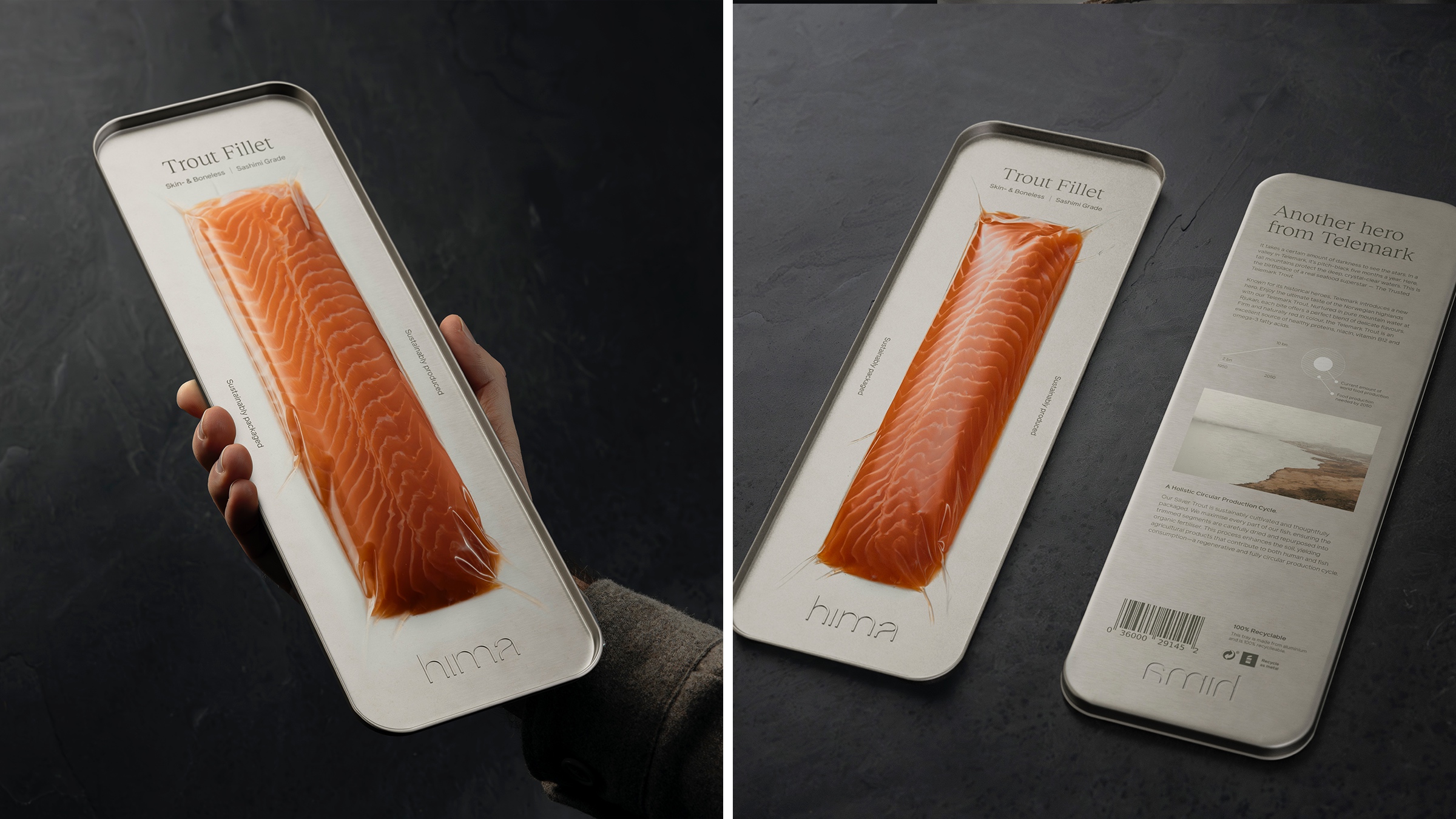This image features two side-by-side photographs of a trout fillet package. The backgrounds of both images are a dark slate gray, creating a stark contrast with the bright packaging. In the left photograph, a man's hand, partially visible with a gray, possibly furry cuffed sleeve, holds the package. The package itself is a sleek, silver stainless steel design, prominently displaying a vacuum-sealed piece of trout fillet. The trout is an orange, fleshy color, marked clearly as H-I-M-A Trout Fillet at the top center of the packaging. 

The right photograph showcases the same trout fillet package, now laying flat on a surface. Next to it is the back of the packaging, which narrates, "Another Hero from Telemark," accompanied by detailed written information about the trout and its preparation. The back also features an image with brown and gray tones, and at the bottom, a barcode is visible alongside an indiscernible number. 

This detailed composition captures both the front and back details of the H-I-M-A Trout Fillet, emphasizing the product's presentation and background information.